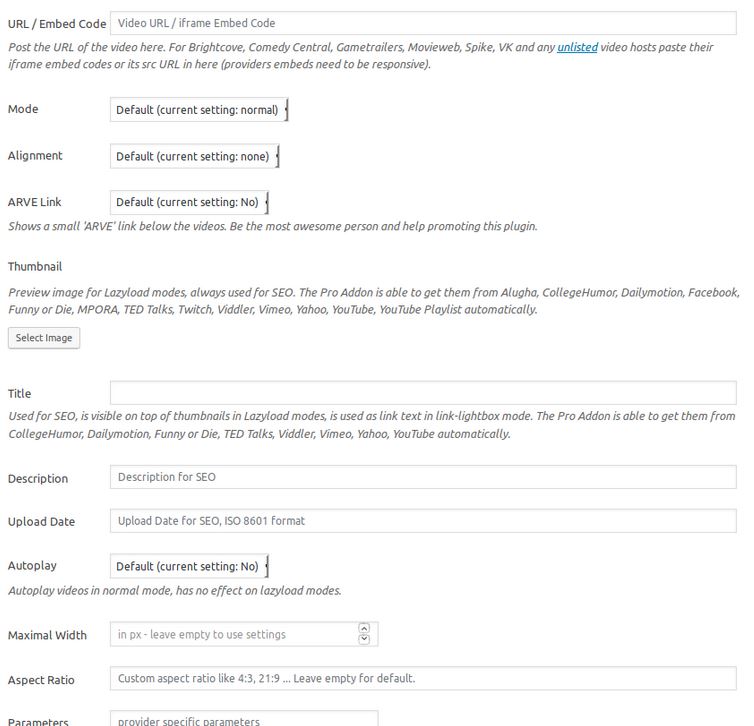Title: Detailed Description of a Web Page Layout for a Video Embedding Plugin

1. **Header Section:**
    - **Primary Heading:** "URL / Embed Code"
    - **Subtext:** "Post the URL of the video here for Brightcove, Comedy Central, Game Trailers, MovieWeb, Spike, VK, and any unlisted video hosts. Paste their iframe embed codes or its SRC URL in here. Providers' embeds need to be responsive."

2. **Input Fields:**
    - A series of text boxes are displayed, each containing prompts for users to input information.

3. **Hyperlink:**
    - A single hyperlink is present in the document, embedded in the word "unlisted." This hyperlink is distinctively colored in blue and underlined.

4. **Settings Section:**
    - **Secondary Heading:** "Mode"
        - **Text Box:** Default setting is "Normal."
    - **Subtext:** Instructions or details about changing the mode setting.
    - **Additional Setting:** "Alignment"
    - **Secondary Heading:** "ARVE Link"
        - **Subtext:** "Show a small ARVE link below the videos. Be the most awesome person to help promote this plugin."

5. **Page Background and Text Color:**
    - The entire web page has a white background.
    - Most of the text on the page is grey.
    - The title and subheadings are in a darker grey, and some subtext is in a lighter grey for distinction.

This web page appears to be a user interface for a plugin that allows users to embed videos from various sources. The detailed layout and prompts are designed to help users input the necessary information for embedding videos effectively while promoting the plugin itself.